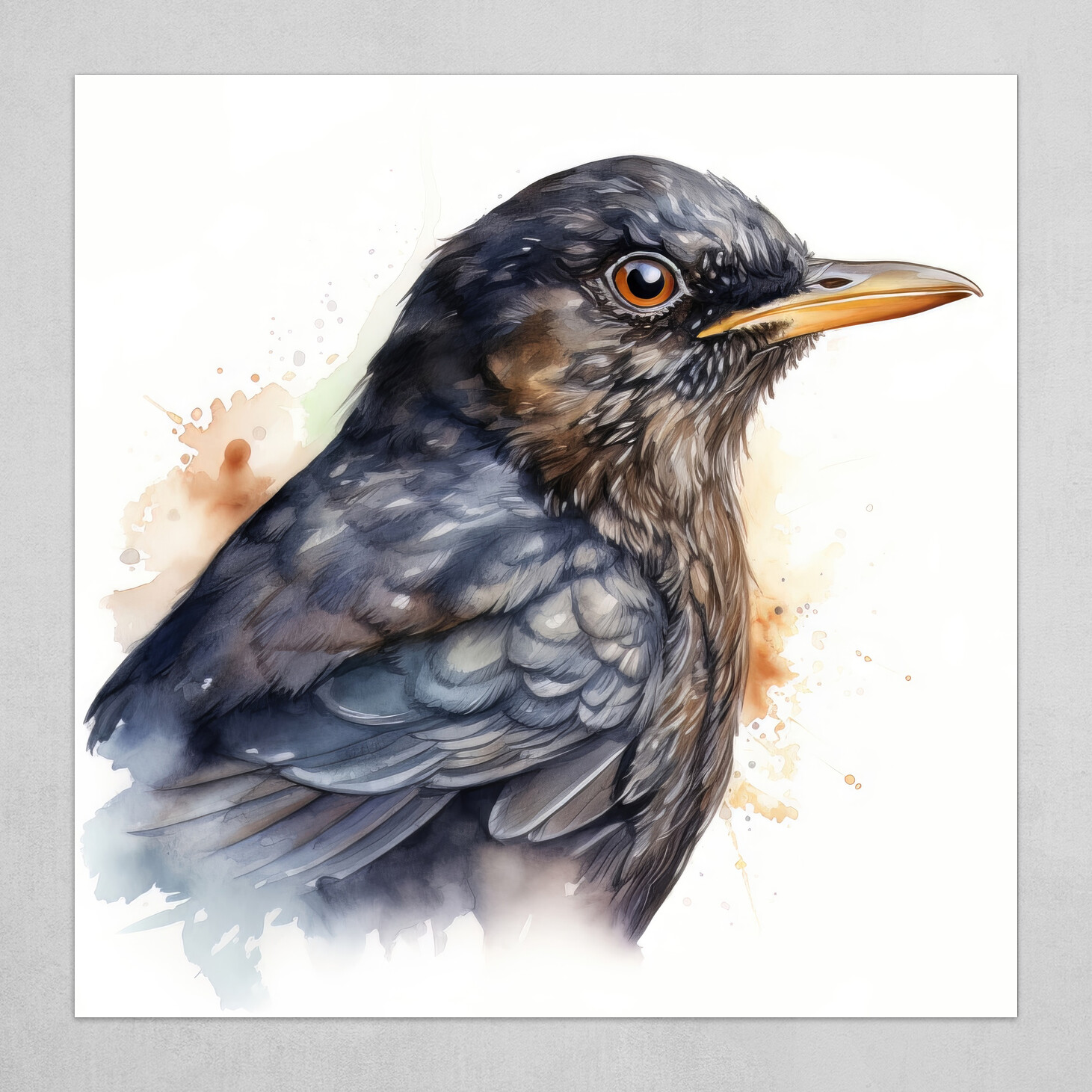This is a highly detailed watercolor painting of a blackbird, depicted in profile from the chest upward. The blackbird's plumage features a nuanced mix of black, blue, and occasional white specks, with a yellow beak and a brown iris encircling a large dark pupil. The bird's head and chest are predominantly black, transitioning into bluish tones toward the back and sides. The background consists of watercolor splotches in shades of brown and green, set against a solid white backdrop. The entire image is framed by a light gray border, adding an elegant touch to the square canvas.